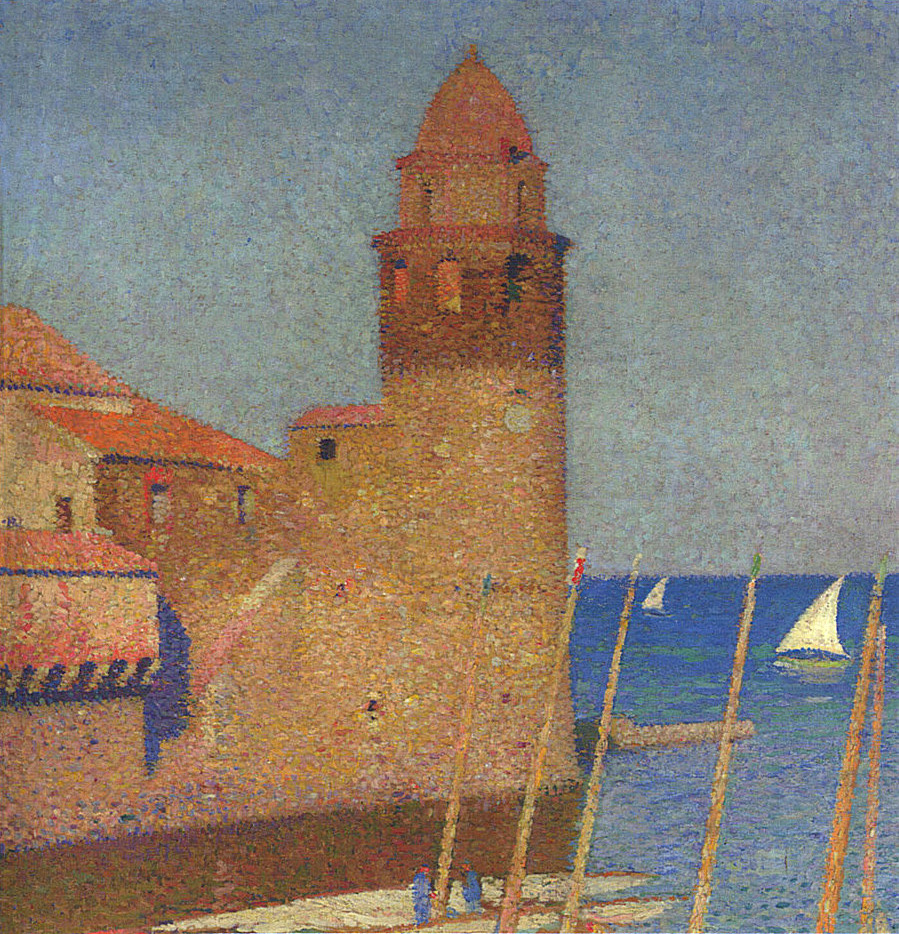The painting is a pointillist-style depiction of a seaside scene dominated by a beige and brown castle with a pointed, red-tiled turret at its center. The castle extends leftwards, featuring a wall that reinforces its fortress-like appearance, reminiscent of architecture found in Spain or Portugal. The composition highlights a tranquil, vivid blue ocean to the right, where two sailboats with white sails glide peacefully. The foreground is adorned with wooden poles rising from the shore, around which two longboats are moored. The sky above is a blend of turquoise and gray, hinting at a possibly approaching storm, further accentuated by the dull, dusty atmosphere. Overall, the painting combines earthy and marine hues, rendered in meticulous, tiny dots that bring depth and texture to the scene.